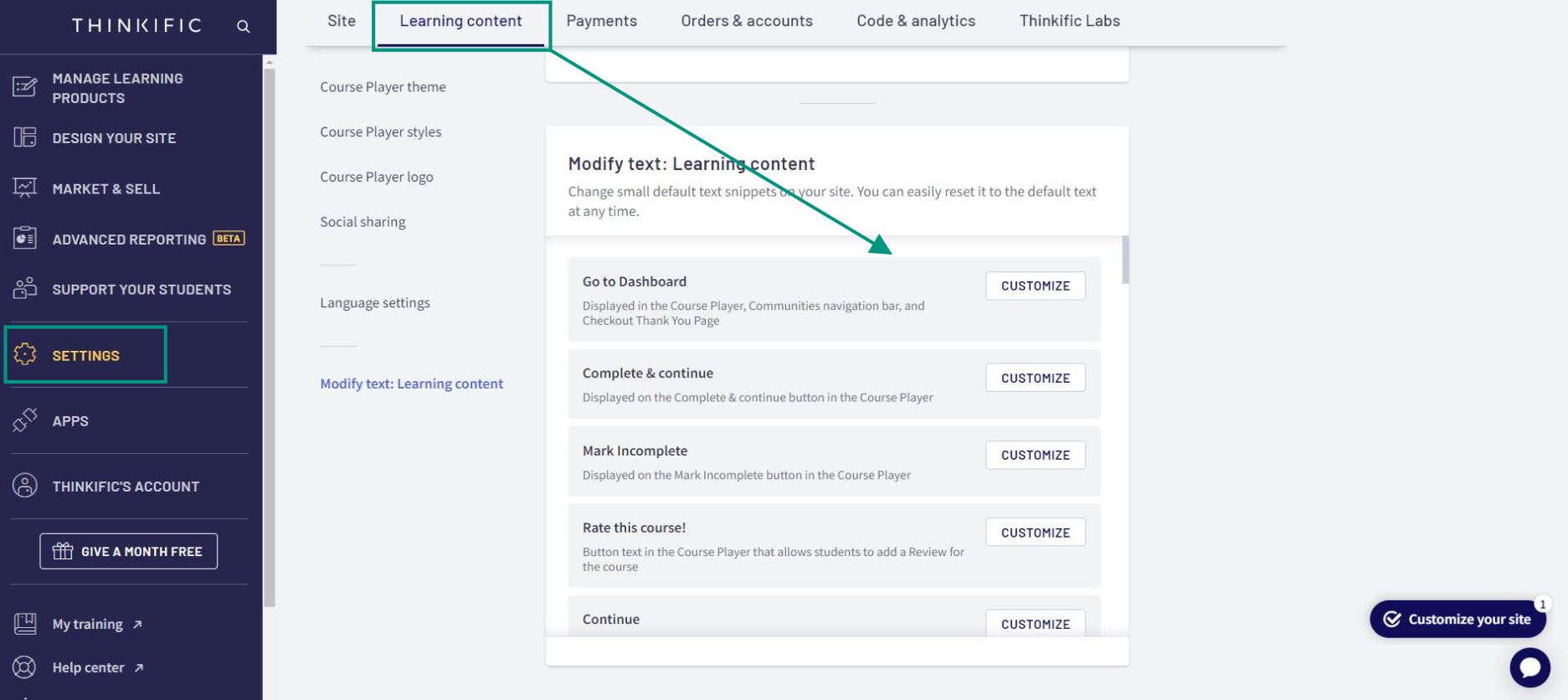The image showcases the user interface of the Thinkific platform, a one-word site for creating and managing online courses. The navigation panel on the left side of the screen features various sections including "Manage Learning Products," "Design Your Site," "Market and Sell," "Advanced Reporting," "Support Your Students," "Settings," "Apps," "Account," "My Training," and "Help Center." External links are also available at the top of the interface.

The user has focused on the "Settings" section, which is highlighted within a box. Inside the "Settings" menu, several options are listed: "Site," "Learning Content," "Payments," "Orders and Accounts," "Code and Analytics," and "Thinkific Labs." The "Learning Content" section is specifically mentioned, indicating that the platform enables users to customize courses and various functionalities to suit their needs. The interface emphasizes course creation and management features, providing a range of tools for a tailored learning experience.